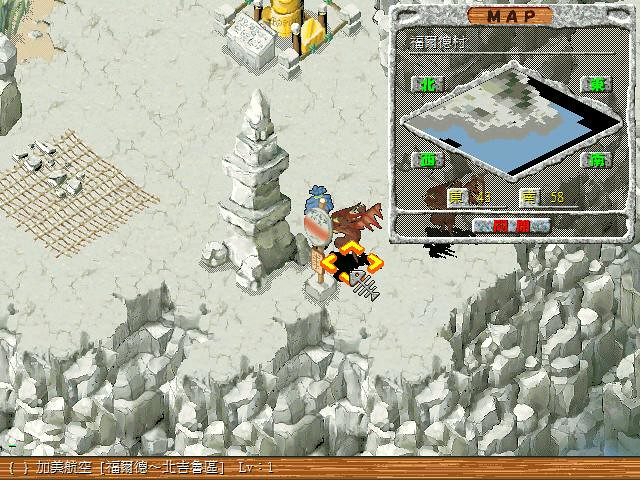This color photograph captures a scene from a computer game characterized by basic graphics and a minimalist design. At the bottom of the screen, a narrow wooden band inscribed with Chinese characters serves as a foundational element. The backdrop features a greyish stone surface with scattered grey rocks in the foreground, creating a rugged environment. In the center of the image stands a squarish tower crowned with a spire, suggesting an architectural focal point. To the left of the tower, a grey mat lies on the ground, adorned with small, indistinct characters.

At the top of the scene, a pile of rubble interspersed with yellow objects adds a sense of disarray and texture. A robot-like game character is positioned beside the tower's spire, adding a touch of animation to the otherwise static background. Surrounding this character are bright yellow arrows pointing in various directions—up, down, right, and left—alongside a cursor, indicating potential navigational options or interactive elements.

On the right-hand side, a square overlay provides an in-game map, replete with various symbols that likely denote points of interest or objectives. Dominating the center of this map is a diamond-shaped element, depicting either a sky with clouds or water near the edge of an island, broadening the scope of the game's environment. The overall scene combines elements of both adventure and strategy within its simplified graphical framework.